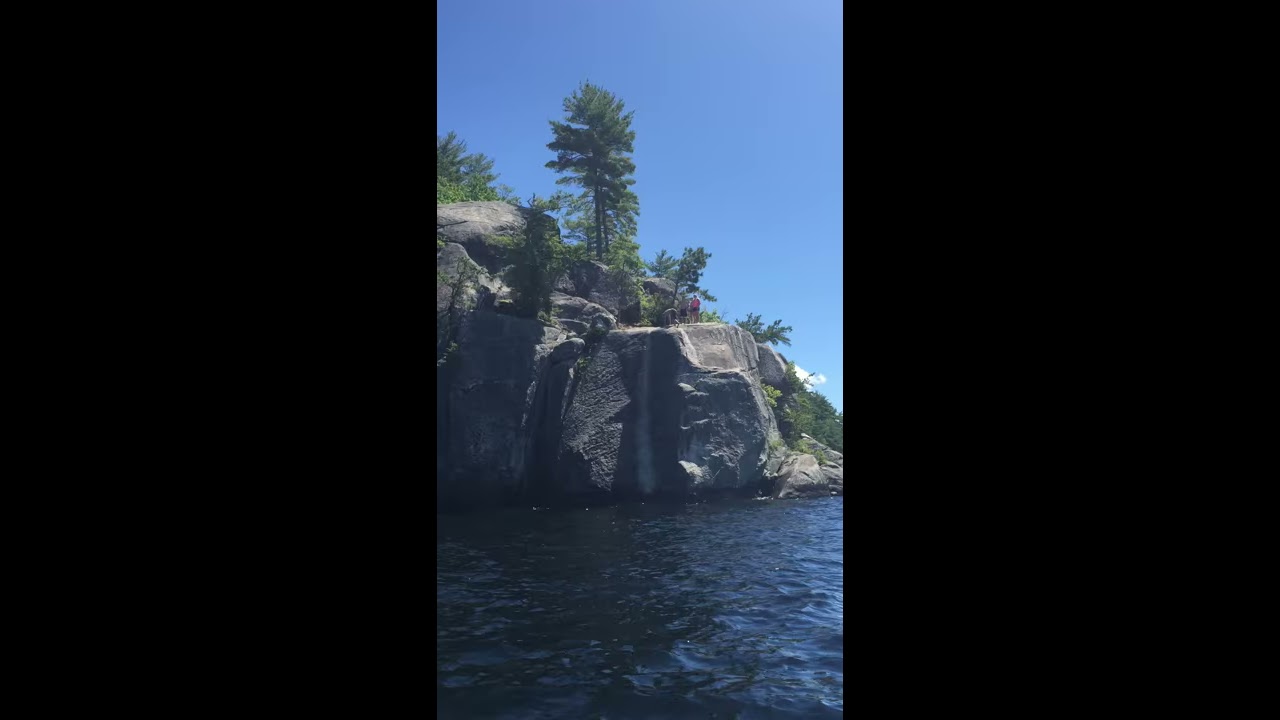This photograph captures a picturesque scene on a clear, beautiful day, featuring a gray, rocky cliff surrounded by deep blue water. Three individuals are standing at the edge of the cliff, seemingly preparing to leap into the serene bay below, set against the backdrop of a vibrant, light-blue sky with a few scattered clouds. The cliff is adorned with lush green trees and bushes, including a prominently centered fir tree with vivid pine needles. The scene radiates tranquility and adventure, capturing the natural beauty and excitement of cliff jumping in a stunningly detailed landscape.